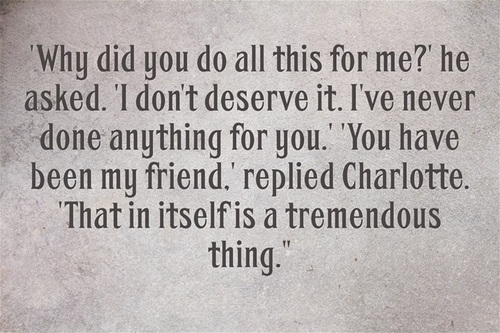The image features a centered, inspirational excerpt from what is likely E.B. White's "Charlotte's Web." The text, in a plain, bookish font, reads: "Why did you do all this for me?" he asked. "I don't deserve it. I've never done anything for you." "You have been my friend," replied Charlotte. "That in itself is a tremendous thing." The background is a speckled, grayish-white, resembling aged, patterned stone, with a darker, opaque area in the upper left corner. The quotation stands out in dark gray or black font, creating a visually simple but poignant presentation, reminiscent of children’s book styling, and often shared as an inspirational quote on social media.